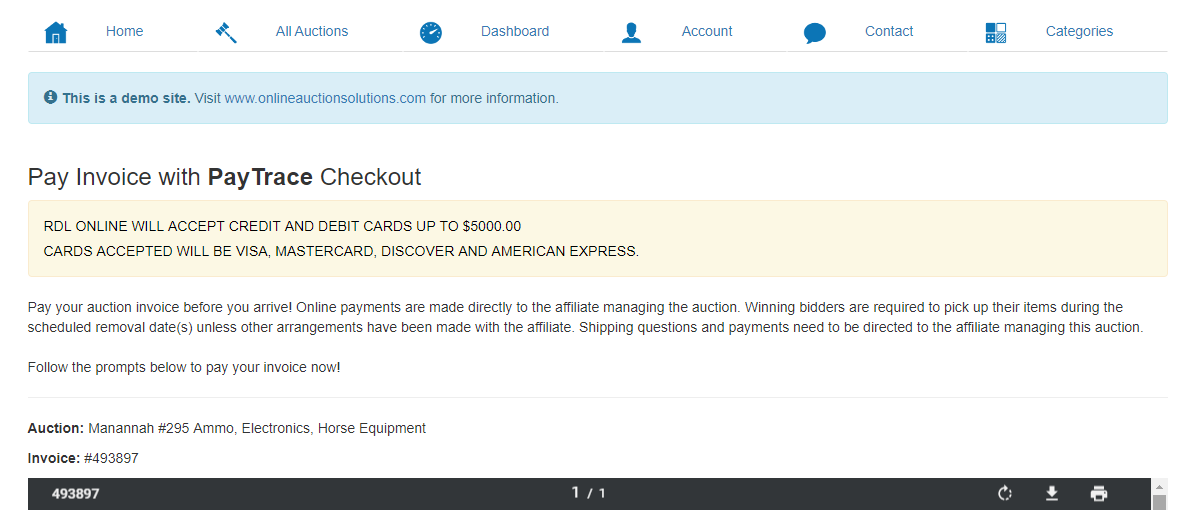Detailed Caption:

The image displays a payment screen from an auction site, specifically a demo page linked to PayTrace Checkout for processing payments. At the top of the page, navigation links are visible, including Home, All Auctions, Dashboard, Account, Contact, and Categories. A notification indicating the demo nature of the site directs users to visit onlineauctionsolutions.com for additional information. The site, still under development, features a predominantly white background with black text.

In the main section of the screen, instructions clarify that RDL Online accepts credit and debit card payments up to $5,000, specifying accepted card types such as Visa and MasterCard. Additional text advises bidders to pay their auction invoices before arrival and notes that online payments go directly to the affiliate managing the auction.

At the bottom, there's further specification about a particular auction event labeled "Auction Mananah #295," listing items such as Ammo, Electronics, and Horse Equipment. "Mananah" appears to denote the auction house location.